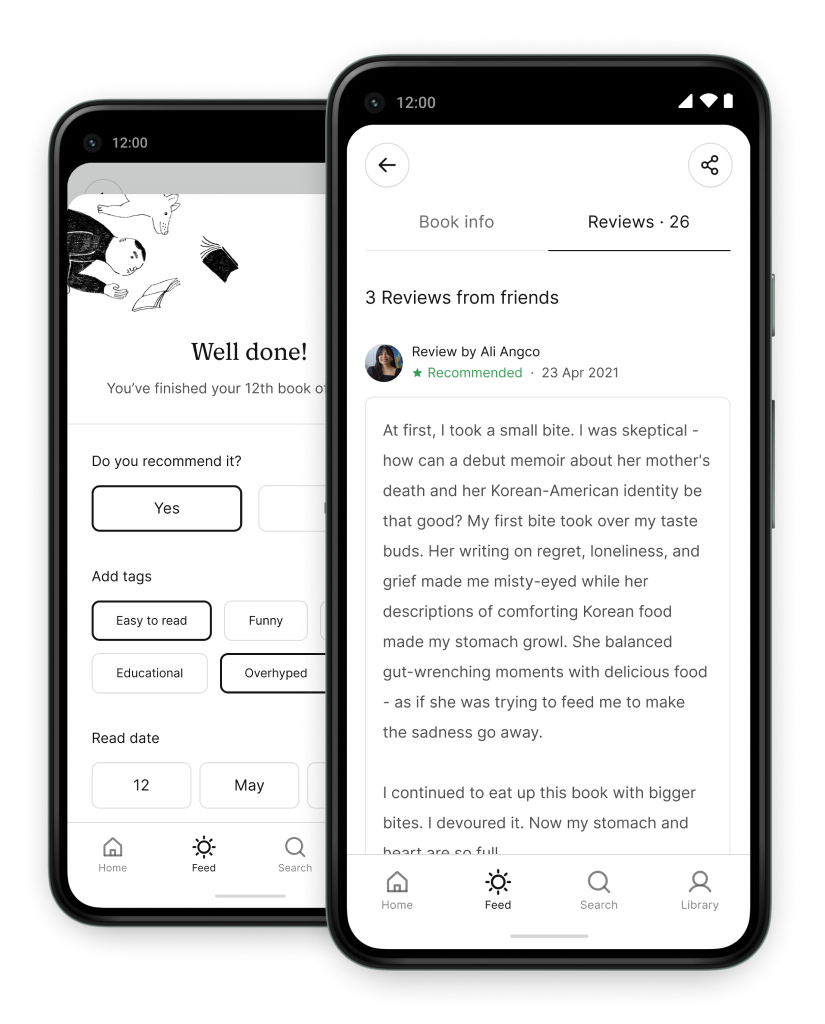A pair of overlapping cell phone screenshots is displayed, with the upper screenshot prominently featured. At the top of this screenshot, the status bar shows the time as 12:00, though it is unclear whether this is AM or PM. Alongside the time, indicators for cell service strength, Wi-Fi signal strength, and battery level are visible. Below the status bar, two main icons are present: a back button on the left and another button to its right. The screen displays a webpage with two main sections: "Book Info" and "Reviews." The "Reviews" section is selected, revealing a total of 26 reviews, including three from friends.

Highlighted within this screen is a recommended review by a user named Allie N. Anko, dated April 23rd, 2021. Allie reflects on a debut memoir that delves into themes of her mother's death and her Korean-American identity. Initially skeptical, Allie describes taking a small bite of the book. The writing, rich with emotions of regret, loneliness, and grief, alongside vivid descriptions of comforting Korean food, made a profound impact. The juxtaposition of gut-wrenching moments with delicious culinary imagery evoked strong emotional and physical responses, likening the author’s intent to feeding the reader to alleviate their sorrow.